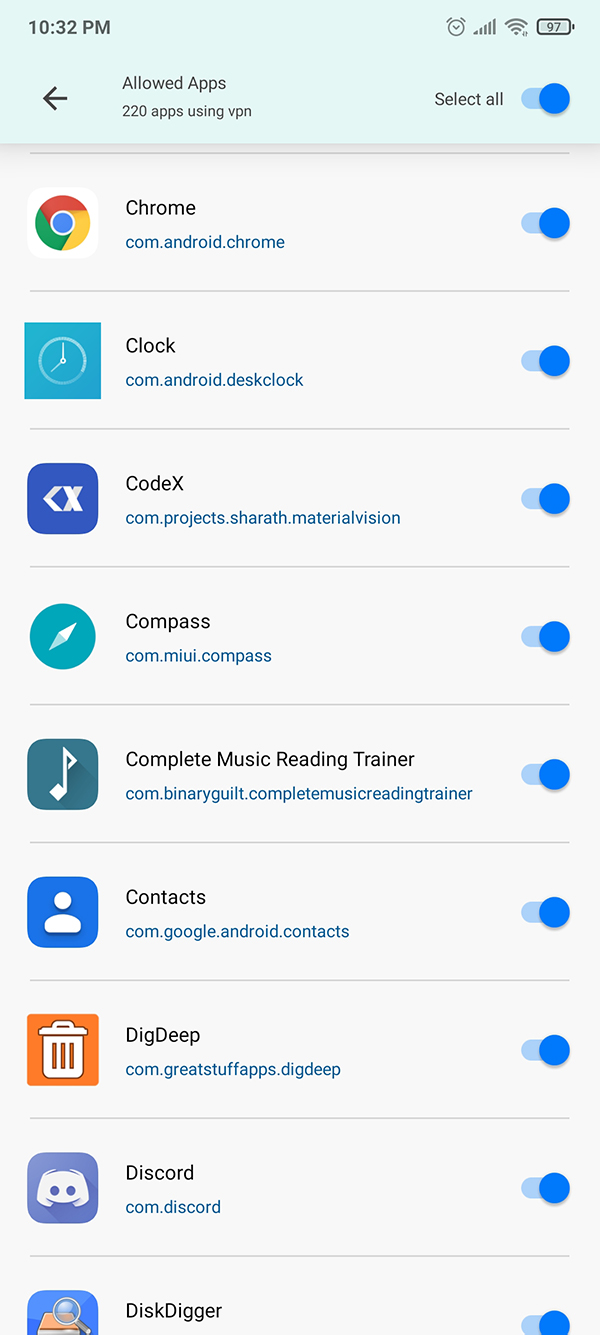This screenshot, captured at 10:32 PM, displays a mobile device with a 97% battery level and a strong signal. At the top of the screen, a green box with the label "Allowed Apps" is visible, indicating that 220 apps are utilizing a VPN, with a "Select All" button activated to the right of the box. The background of the screen is predominantly white, and all toggle switches for the listed apps are set to "On." 

Notable apps shown include Chrome, Clock, CodeX, Compass, Complete Music Reading Trainer (identified also by its package name BinaryGuilt.CompleteMusicReadingTrainer), Contacts, Dig Deep, Discord, and Disk Digger. This selection represents a fraction of the total apps managed under VPN settings in the device.